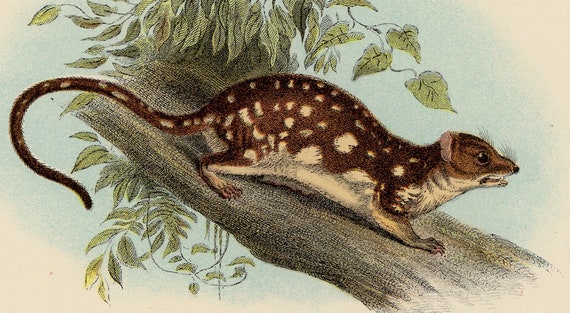This image is a detailed hand-drawn picture featuring a four-legged animal perched on a robust tree branch. The animal, seen from the side, has a primarily brown body with cream-colored spots and a cream underside. Its long tail and slightly open mouth give it an alert, possibly aggressive appearance, as it looks towards the right. The creature, which resembles a rat but may be a ferret, mongoose, or badger, also has black eyes and whiskers. The setting includes several green leaves on the branch and a light blue background. The drawing is executed with colored pencils, showcasing soft and delicate shading, especially on the bark of the tree. The image itself has a border with white edges and a circular blue hue in the middle, enhancing its detailed artistry.